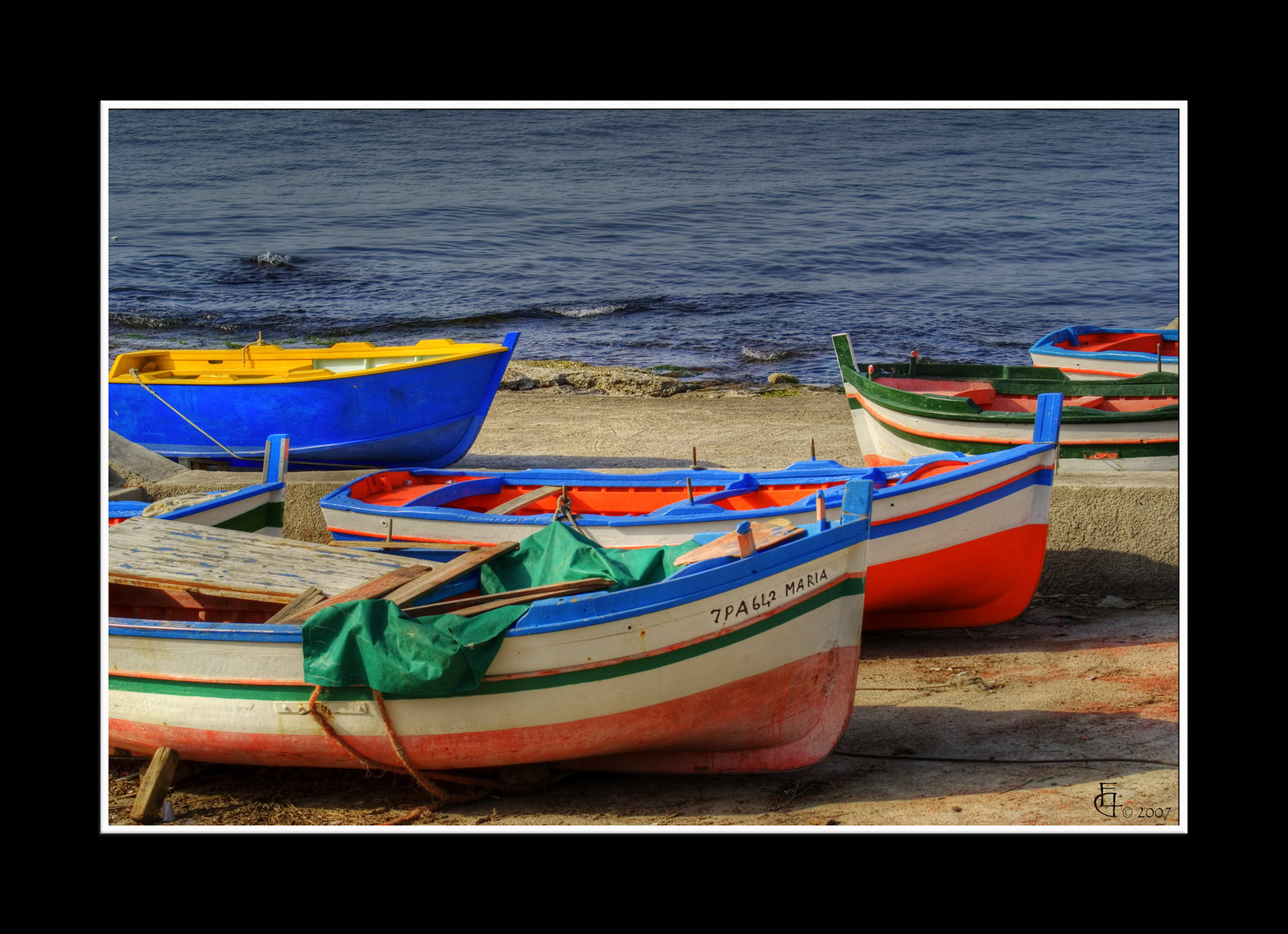This image captures an outdoor scene of five small fishing canoes arranged on a sandy beach that borders a lake. The picture features a black outer border and a narrower white inner border. At the top of the image, there's blue water with ripples and a tiny wave near the center. The shoreline transitions into sand, which is piled up in various areas.

On the left side of the image, a blue canoe is slightly separated from the others. In the middle, two canoes with red bottoms and beige stripes dominate the foreground. One of these canoes has additional green, orange, and blue stripes, and a green bag can be seen inside it. These boats are vividly colored, with combinations such as blue, white, orange, red, and green. Distinctively, the front canoe displays the text "7 PA 662 Maria."

Finally, on the right side of the image, a watermark reading "2007" is visible, indicating perhaps the year the photograph was taken. These small fishing canoes are designed to hold up to four people, and they can easily be pulled out of the water.